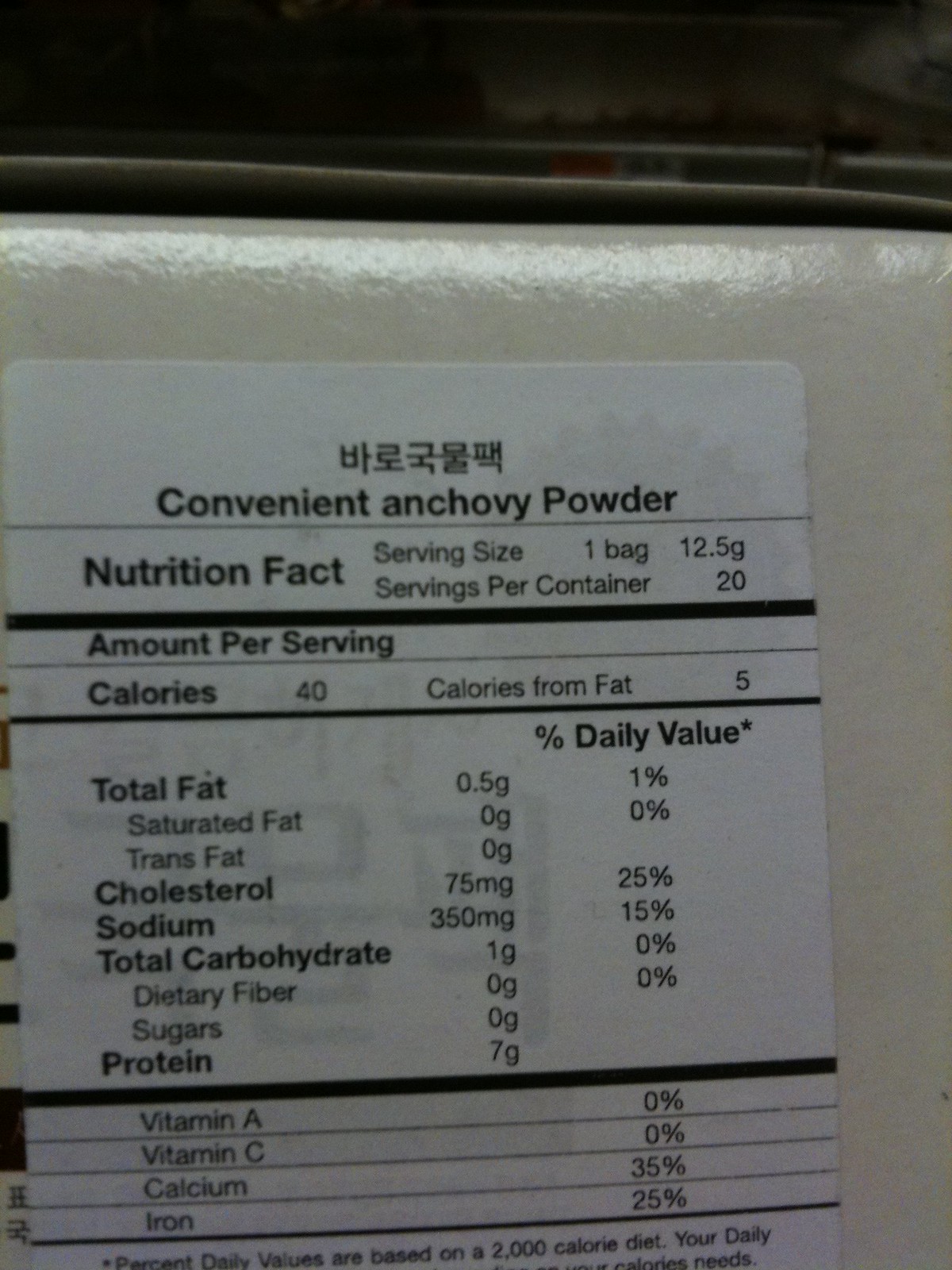This is an image of a label detailing nutritional information for a product labeled "Convenient Anchovy Powder," accompanied by Asian script presumably clarifying the product name. The label prominently displays "Nutrition Facts" with sections below specifying serving size and servings per container, followed by numerical values. The nutritional breakdown includes calorie count, calories from fat, total fat, saturated fat, trans fat, cholesterol, sodium, total carbohydrates, dietary fiber, and other relevant nutritional metrics. The label appears adhered to the back of a white object, likely the product packaging.